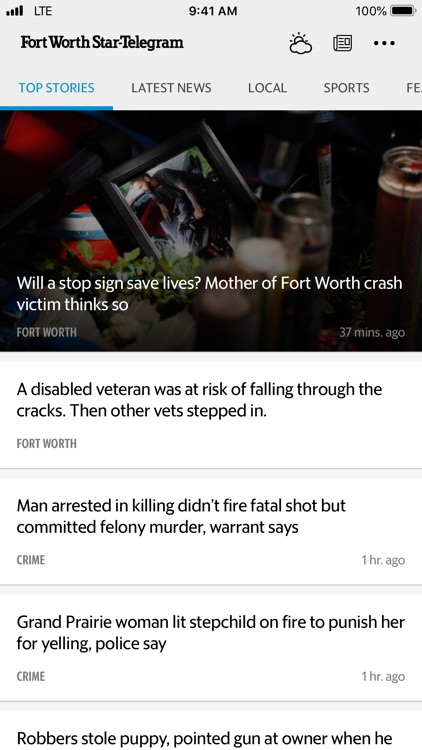Screenshot of a mobile phone's display at 9:41 AM. The status bar at the top shows full mobile signal with LTE on the left, the time in the center, and a fully charged battery icon with "100%" on the right. Directly below, in black font, it reads "Fort Worth Star Telegram," accompanied by a weather icon showing a sun partially obscured by a cloud, a newspaper icon, and three horizontal black dots.

The main section presents various categories of the website - Top Stories, Latest News, Locals, Sports, and Fields. The "Top Stories" section is currently selected. The leading story, posted 37 minutes ago, features an image of a framed photograph with candles placed before it. The photo within the frame shows a man dressed in a weather jacket. The headline reads: "Will a stop sign save lives? Mother of Fort Worth crash victim thinks so." Below this, another headline reports, "A disabled veteran was at risk of falling through the cracks. Then other vets stepped in."